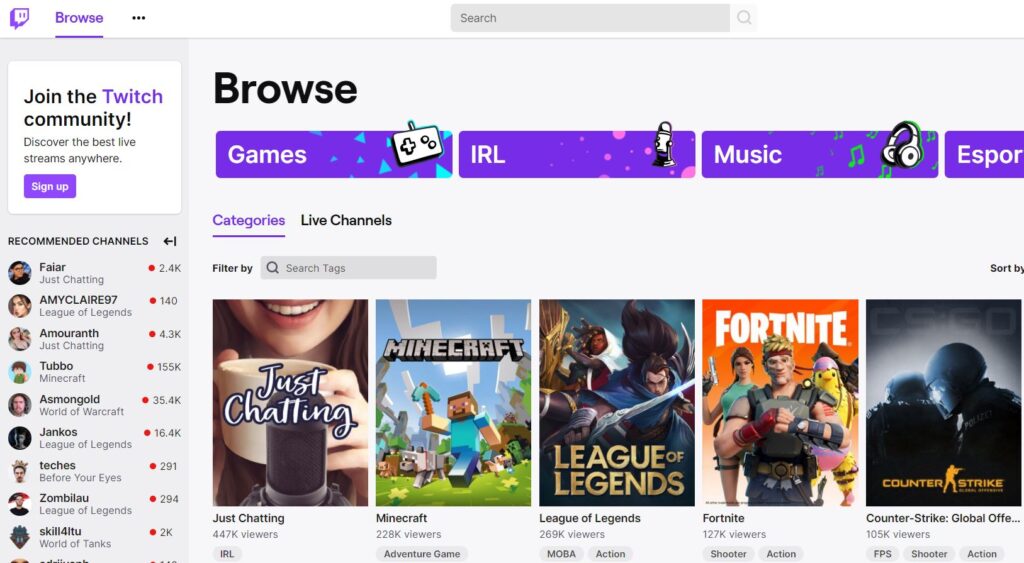This is the launch page for Twitch's "Browse" option. In the upper left corner, there is the prominent purple Twitch icon, which resembles two chat boxes stacked on top of each other, with the inner chat box containing two small dot "eyes." Adjacent to the icon, there's an underlined "Browse" hyperlink, indicating that the user is currently on the Browse page. To the right of this, there is a hamburger menu, followed by a search bar with a magnifying glass icon.

Directly beneath this section, the word "Browse" is displayed in black lettering. Below it, there is a purple background strip with white text labels for "Games," "IRL," "Music," and "S4," accompanied by respective icons—a controller, a microphone, and headphones. Further down, the underlined word "Categories" indicates the section being viewed, with "Live Channels" as an option to the right.

The filter section, labeled "Filter by" with a magnifying glass icon, allows users to search for specific tags. Following this, popular categories such as "Just Chatting," "Minecraft," "League of Legends," "Fortnite," and "Counter-Strike: Global Offensive" are displayed, each represented by relevant thumbnail images.

On the left side of the page, a prompt invites users to join the Twitch community with the message, "Discover the best live streams anywhere," and offers a purple "Sign Up" button. Below this area, there is a "Recommended Channels" section listing nine visible channels that Twitch suggests, each channel name accompanied by the current viewer count displayed to the right.